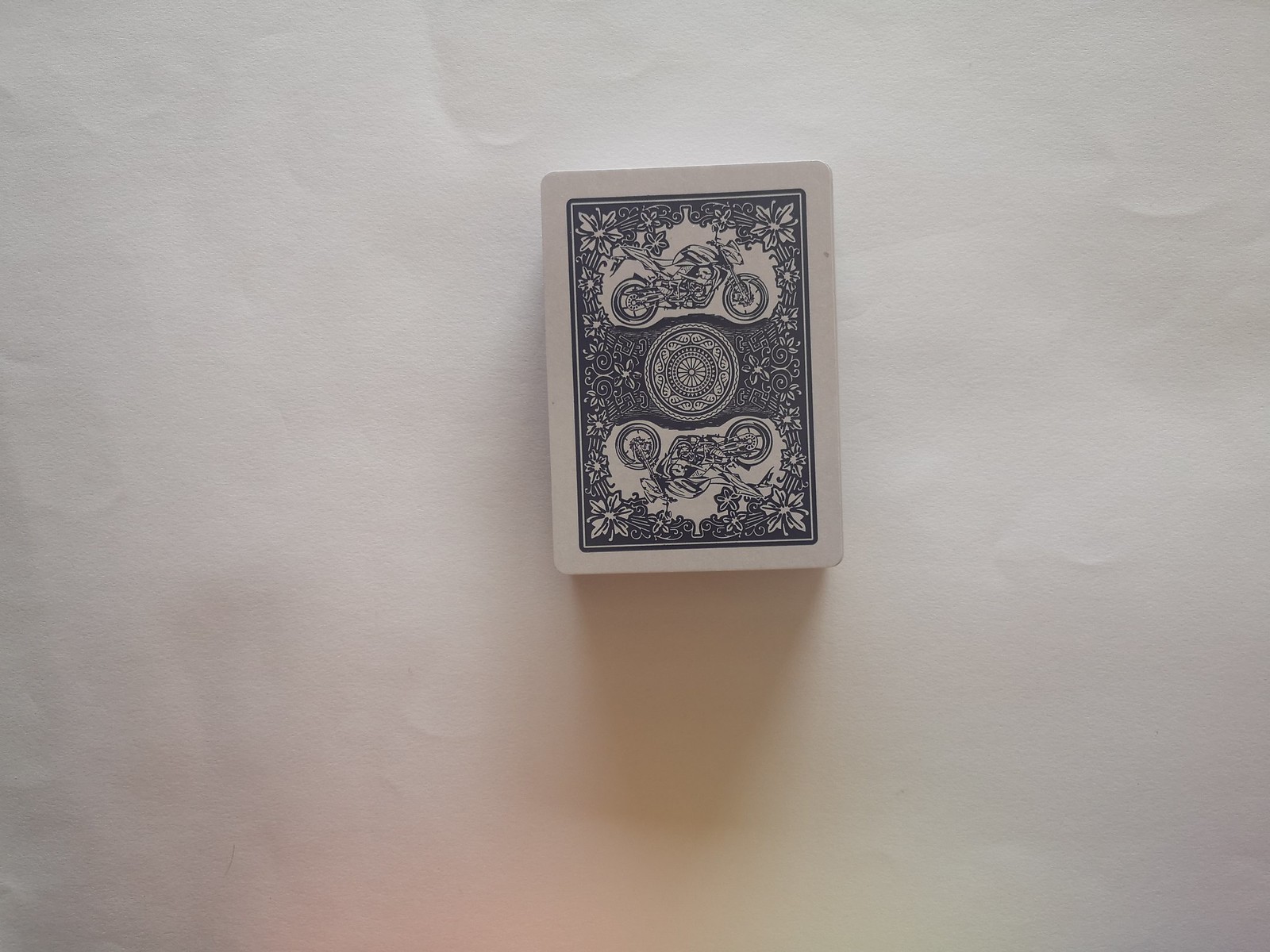A deck of cards rests on a white piece of paper that serves as the background of this photograph. The paper shows subtle signs of having been flexed, creating a loopy mark that adds texture to an otherwise plain surface. Positioned slightly askew from a perfectly vertical orientation, the deck is aligned more towards the left, causing a touch of visual dissonance. Shadows cast by the deck fall to the bottom left, extending towards the edge of the paper, which is laid out in a landscape orientation.

The deck itself features a fascinating design: a Kawasaki motorcycle rendered in a low, sleek style appears prominently along with a traditional floral pattern. These elements are accented with a mandala-type design centrally placed, offering a blend of modern and classical aesthetics. The cards are framed by a white border and feature a color scheme of blue and white. The blue, however, is not a vibrant hue but rather a muted, slate blue that lends a subdued elegance to the deck.